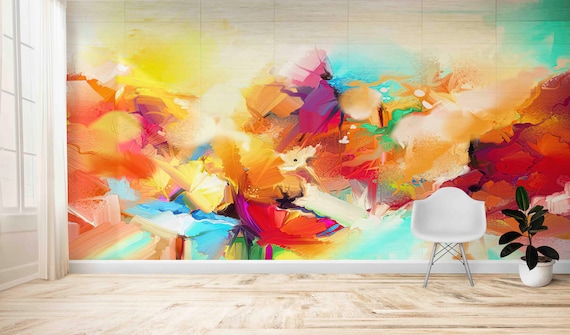In this image, a vivid mural featuring an abstract, watercolor-style painting adorned with various colors, including dominant shades of red, yellow, orange, blue, and purple, decorates the wall. The background of the mural is a mix of light blue and white, intensifying the bursts of colors that merge into brush strokes and flower-like impressions. On the left side of the mural, orange and dark orange flowers blend into a sea of white, while the center showcases striking red and purple flowers extending towards the top. Towards the upper right corner, swathes of yellow, orange, red, and light blue paint create an airy, almost ethereal visual effect.

In front of this mural is a sleek white plastic chair with contrasting silver metal legs. To the right of the chair stands a potted green plant in a chic white planter. The room boasts a sophisticated light brown and white marbled floor, enhancing the elegance of the minimalist decor. To the left of the composition, a large window with sheer white drapery allows natural light to flood the space, illuminating the room and highlighting the intricate details of the artwork. The overall scene is a harmonious blend of modern furniture and colorful, artistic expression, captured within an interior setting.